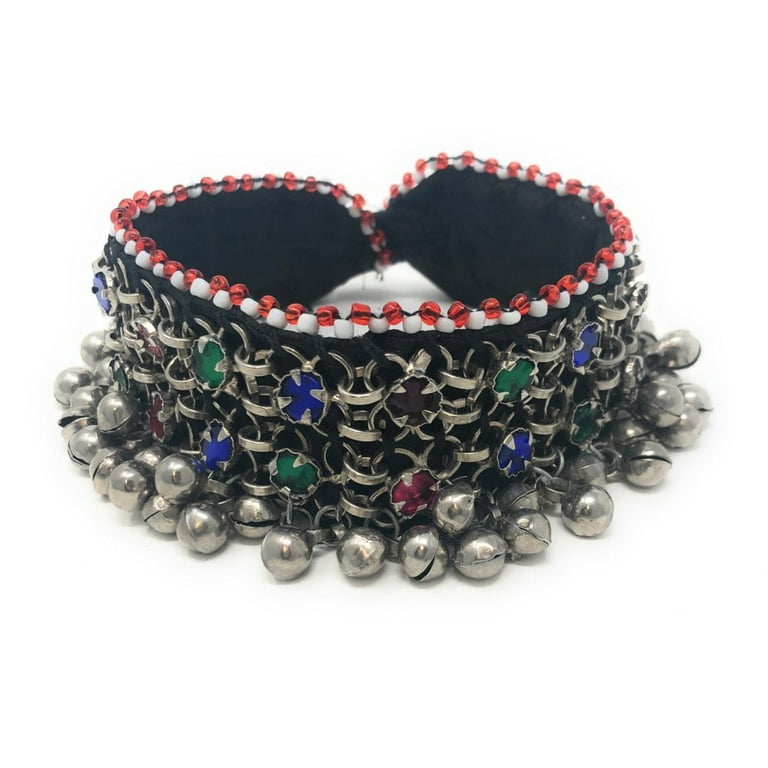The image depicts an intricately crafted piece of jewelry, predominantly black, and possibly serving as a bracelet, anklet, or even a choker necklace. The main body appears to be a loop of chain mail, interspersed with occasional semi-precious stones in colors like green, red, and blue, set in four-pronged holders. These metal rings are linked together and intricately laced, framed by a felt or cloth liner to prevent scratching. At the top of the jewelry piece, alternating red and white beads add a touch of color. The bottom edge is adorned with a row of small silver bells that resemble sleigh bells. The entire item is displayed against a featureless white background, enhancing its detailed craftsmanship and hinting at a handmade design.